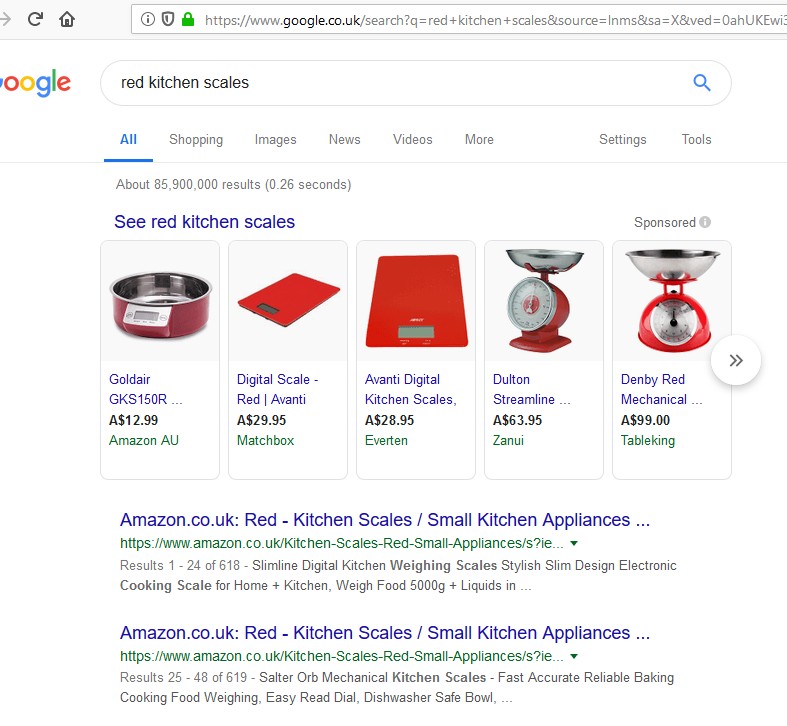This image is a cropped screenshot of a Google search results page for the query "Red Kitchen Scales." The top section shows a thin gray search bar above a white search bar with the partially visible Google logo on a google.co.uk domain, where the initial 'G' is cut off. The query "Red Kitchen Scales" is typed into the search bar, and the "All" tab is selected among the options: All, Shopping, Images, News, Videos, and More. The search returned approximately 85,900,000 results in 0.26 seconds.

Below this is a blue link text labeled "See Red Kitchen Scales," followed by six advertisements showcasing various red kitchen scales of different designs. 

1. **Gold Air GKS-150R** - This resembles a red pot and is priced at £12.99, available on Amazon EU.
2. **Digital Scale Red Avanti** - A red pad-like scale priced at $29.95, offered by Smashbox.
3. **Avanti Digital Kitchen Scales** - Another red pad scale, priced at $28.95, provided by Everton.
4. **Dalton Streamline** - A red scale with a silver bowl, priced at $63.95, available on Zenui.
5. **Denby Red Mechanical** - Another red scale with a silver bowl, priced at $99, available at Table King.

Additional search options from Amazon.co.uk featuring red kitchen scales are shown below the advertisements.